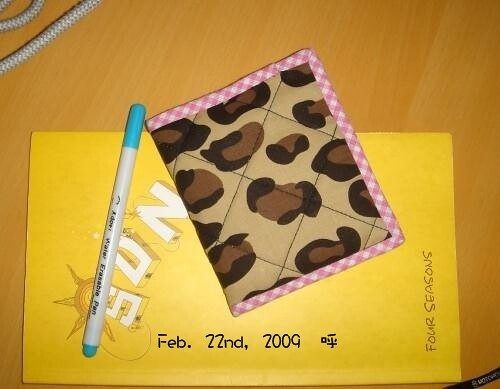The image illustrates a letter-sized, bright yellow package or folder resting on an orange wooden surface with the text "Sun" written in blocky white letters at the top left, accompanied by a small artistic sun icon. Across the middle is the date, "February 22nd, 2009," written in a thicker black marker or edited on, with a possible additional character next to the year that resembles an Asian symbol. Vertically on the right-hand side, the words "Four Seasons" are written in pen. Nestled on the upper left side of this folder is a pin with a turquoise cap, and to its right is a large piece of fabric. This fabric has a pink plaid border and a brown, leopard print inside, and appears to be a thin, thready material used for handling pans, similar to a mitten but not quite one. Additionally, in the upper left corner of the image, there is a glimpse of a phone cord trailing off the screen.